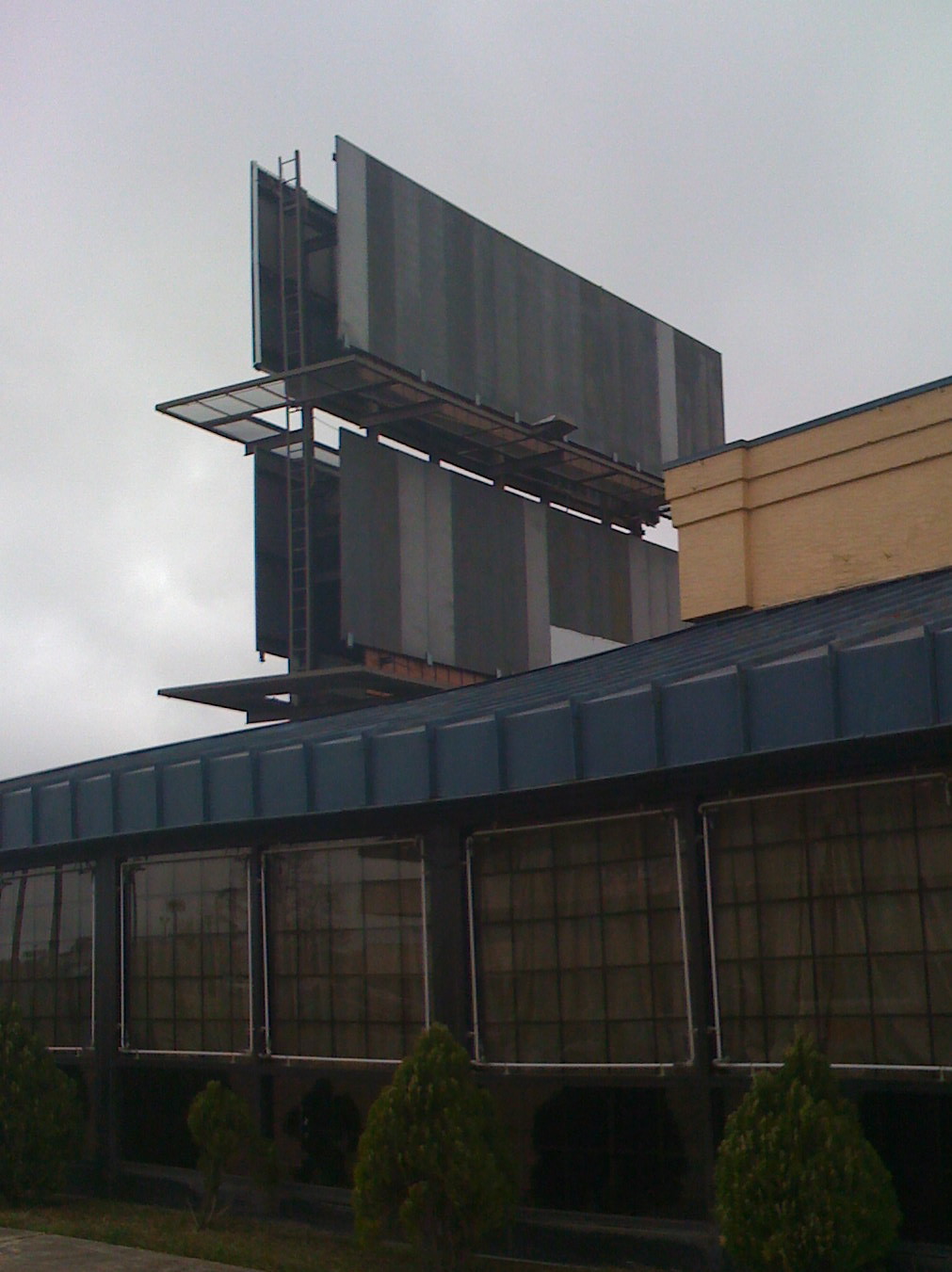The image portrays the side view of a one-story building with the back ends of two rectangular, gray billboard signs positioned above it. In the bottom left corner, a strip of gray sidewalk is visible, immediately bordered by a stretch of green grass adorned with four young, green trees. The building itself has a dark blue upper and lower frame and features five square windows with intricate brown patterns of small squares. The roof is tan on the right side, contrasting with the gray billboards on the left. The sky in the background is a mix of light gray and white hues, adding a soft, overcast ambiance to the scene.